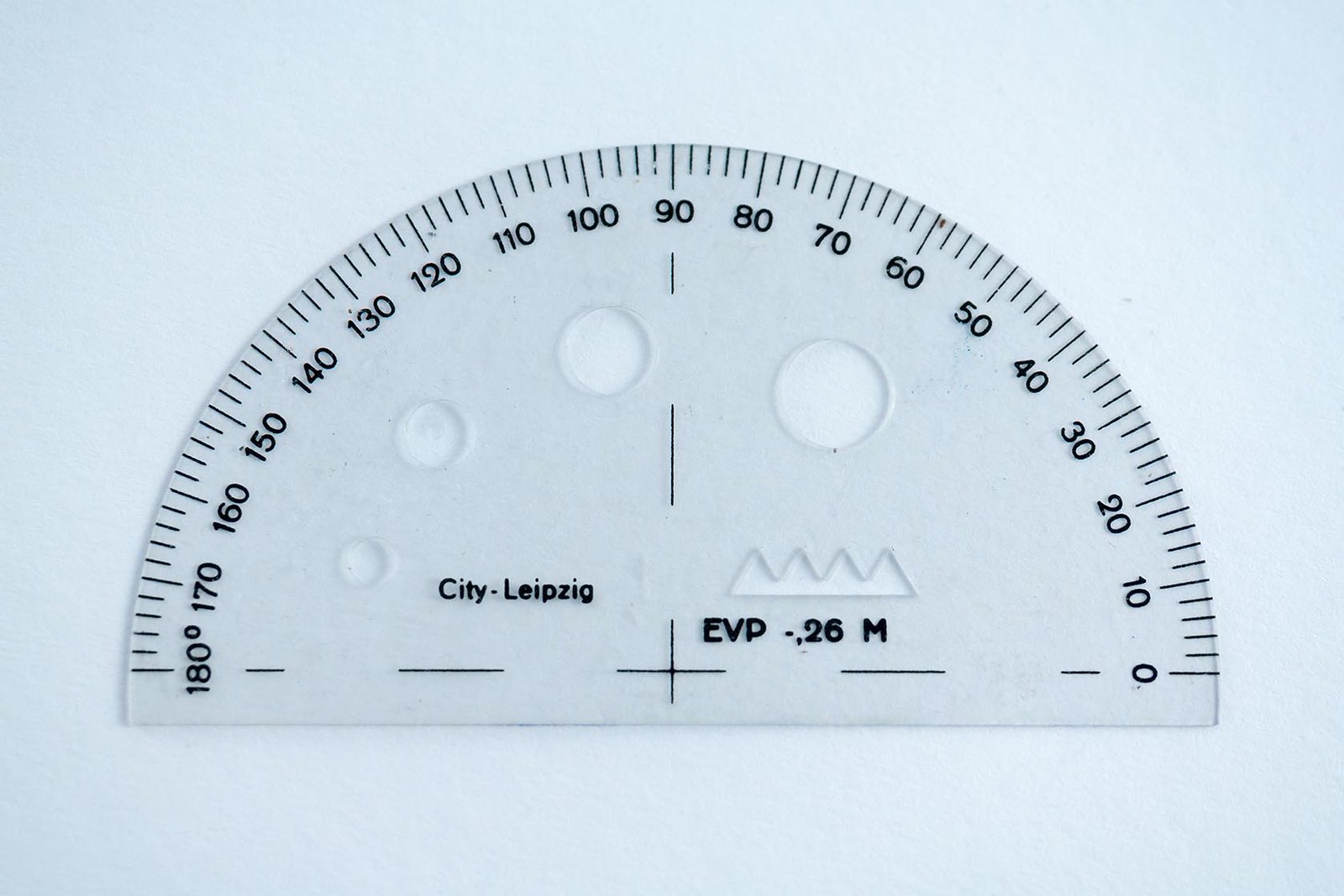The horizontally rectangular image depicts a realistic photograph of a measuring tool, likely a protractor, set against a simplistic, light blue background that appears to be either a table or a piece of paper. The protractor is made of clear plastic and represents the top half of a circle, flat in form, with black markings etched along its outer curved edge. 

The markings are numerically indicated from 180 degrees on the far left, descending clockwise in 10-degree increments (170, 160, 150, and so forth) until reaching 0 degrees at the bottom right. These degree markings are neatly organized with small dash marks at each degree interval.

Within the protractor, four circular cutouts progressively vary in size from left to right: a small circle, a medium circle, a larger circle, and the largest circle on the far right. Below the largest cutout is a series of four small, black triangles pointing upwards, resembling mountain peaks.

Additional text is located on the left side of the protractor, reading "City Leipzig" in black. Beneath the four triangle icons, the text "EVP negative 0.26M" is printed in similarly black lettering.